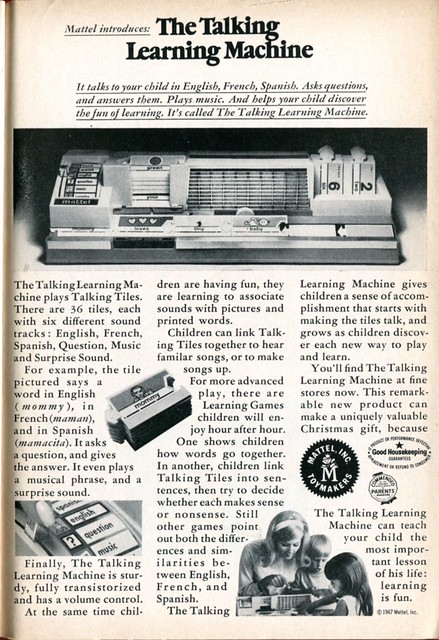This vintage advertisement showcases Mattel's 1967 breakthrough educational toy, the Talking Learning Machine. Dominating the upper section of the ad, the headline reads: "Mattel Introduces the Talking Learning Machine," followed by a description emphasizing its capabilities: it speaks to children in English, French, and Spanish, asks and answers questions, plays music, and makes learning enjoyable. The machine itself, depicted as a large device placed on a table, is complemented by detailed text explaining its features and benefits.

The central image of the Talking Learning Machine is visually framed by three columns of text below it. The first column explains that the machine uses 36 talking tiles, each containing six soundtracks in multiple languages. An example provided is a tile that pronounces the word 'mommy' in English, 'maman' in French, and 'mamacita' in Spanish. Additionally, the tiles include questions, answers, music, and surprise sounds. 

The middle column highlights how children can engage with the machine by linking tiles to form sentences or songs, facilitating advanced play that includes learning games. These activities help children recognize word association, sentence structure, and language differences while reinforcing the idea that learning is fun. 

The third column underscores the machine's sturdiness, full transistorization, and volume control, ensuring it is both durable and adaptable to different play environments. The advertisement concludes by positioning the Talking Learning Machine as an ideal Christmas gift due to its unique educational value. The bottom of the ad features logos from Good Housekeeping, Mattel, Inc., Toymakers, and the copyright notice from 1967.

The advertisement's color scheme is composed of blacks, whites, grays, and a pale off-yellow, contributing to its vintage aesthetic.